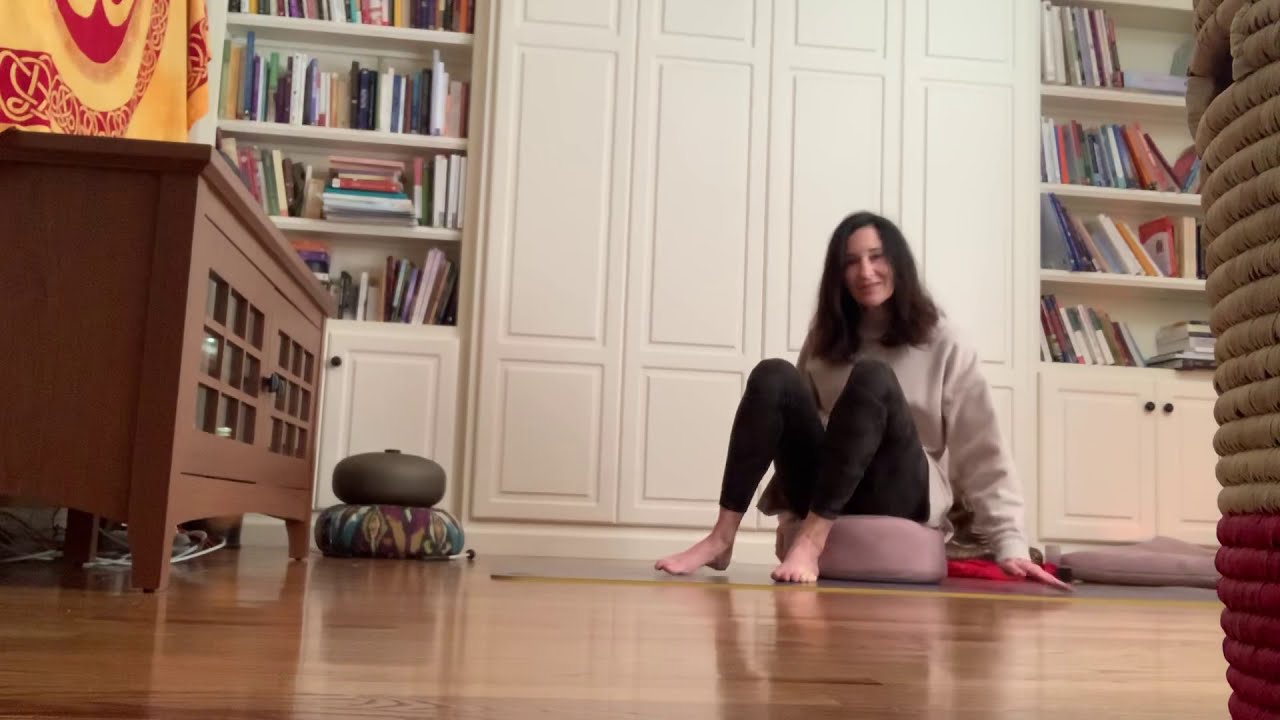This photograph, taken from floor level in a cozy living room setting, captures a woman seated on a pink floor cushion at the center of the frame. The backdrop features built-in white bookcases brimming with various books. To the left, there is a darker wood-finished entertainment center with two glass doors. The woman, appearing to be in her 40s or early 50s, has long, slightly wavy brown hair that falls just past her shoulders. She is dressed in a tan sweatshirt paired with black leggings and is barefoot. Her posture is relaxed, with her knees drawn up to her chest and her hands resting on the floor. She smiles warmly at the camera. Also seen in the image are additional cushions, including a gray one atop a multicolored pad to her right and a flat cushion on the left. A metal bowl rests on one of the cushions. On the far right, a wicker basket extends from top to bottom of the frame. Additional details include a wooden chest with drawers to the left of the basket and some red and orange drapery hanging in the upper left corner of the room.